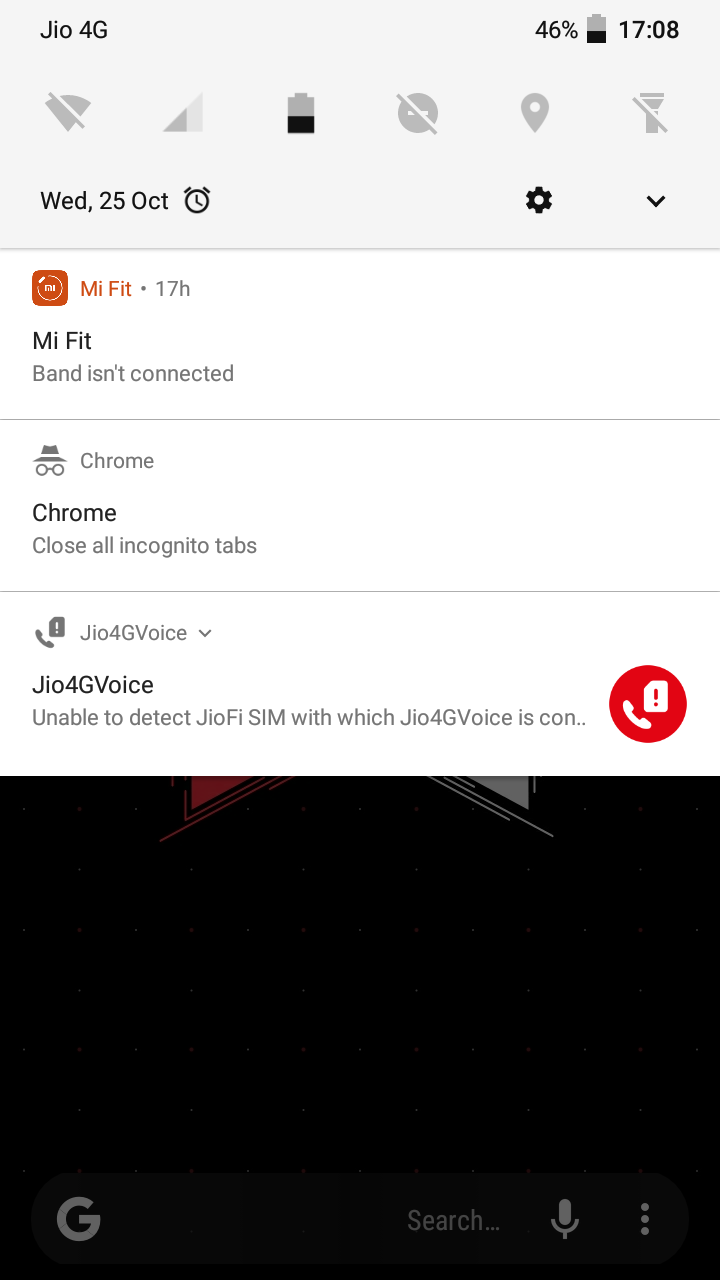This image is a screenshot from a smartphone's settings area. At the top right, the time is displayed as 17:08. Adjacent to this, there is a vertically-oriented battery icon, indicating that the battery is 46% charged. To the left of the time, "GIO" and "4G" are shown, indicating the network provider and connectivity status. Below these, a series of small, grayish icons depict the Wi-Fi signal, phone signal strength, battery status, a "do not disturb" symbol, a location/map pin, and a flashlight.

On the far left beneath this row, the date is displayed as "Wednesday, 25 October." To the right, a gear icon accompanied by a downward arrow is seen, indicating a settings menu or additional options.

The middle of the image contains several sections. The top section features "MeFit" in orange lettering next to the MeFit logo, and below it, the message "MeFit band isn't connected" is displayed, suggesting that the MeFit fitness band is not currently linked to the device. The next section below this states, "Chrome close all incognito tabs," presumably a recent notification or command. The final section at the bottom of the screen indicates "GIO 4G voice," likely referring to the current network service status.